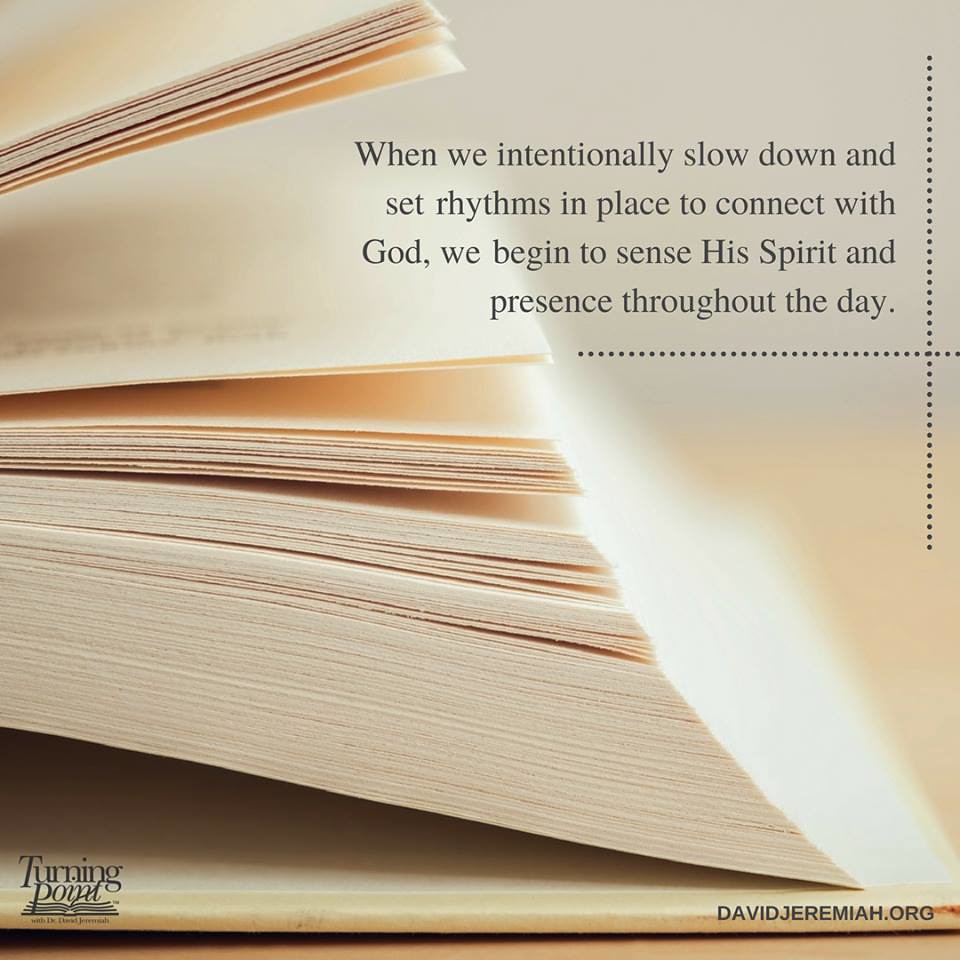The image features an open hardcover book with beige pages, viewed from the bottom left corner, where the outer edges of the pages and the light yellow-beige cover are visible. Superimposed above the book is a quote in gray font that reads, "When we intentionally slow down and set rhythms in place to connect with God, we begin to sense His spirit and presence throughout the day." This text is accentuated with dotted lines, adding a serene and structured visual effect. The lower right corner of the image is marked with the text “davidjeremiah.org” in uppercase black writing, while the bottom left corner bears the logo and text "Turning Point with Dr. David Jeremiah." The overall ambiance of the image is calming, with bright daylight filtering in, contributing to a peaceful and reflective atmosphere meant to evoke a sense of spiritual connection.